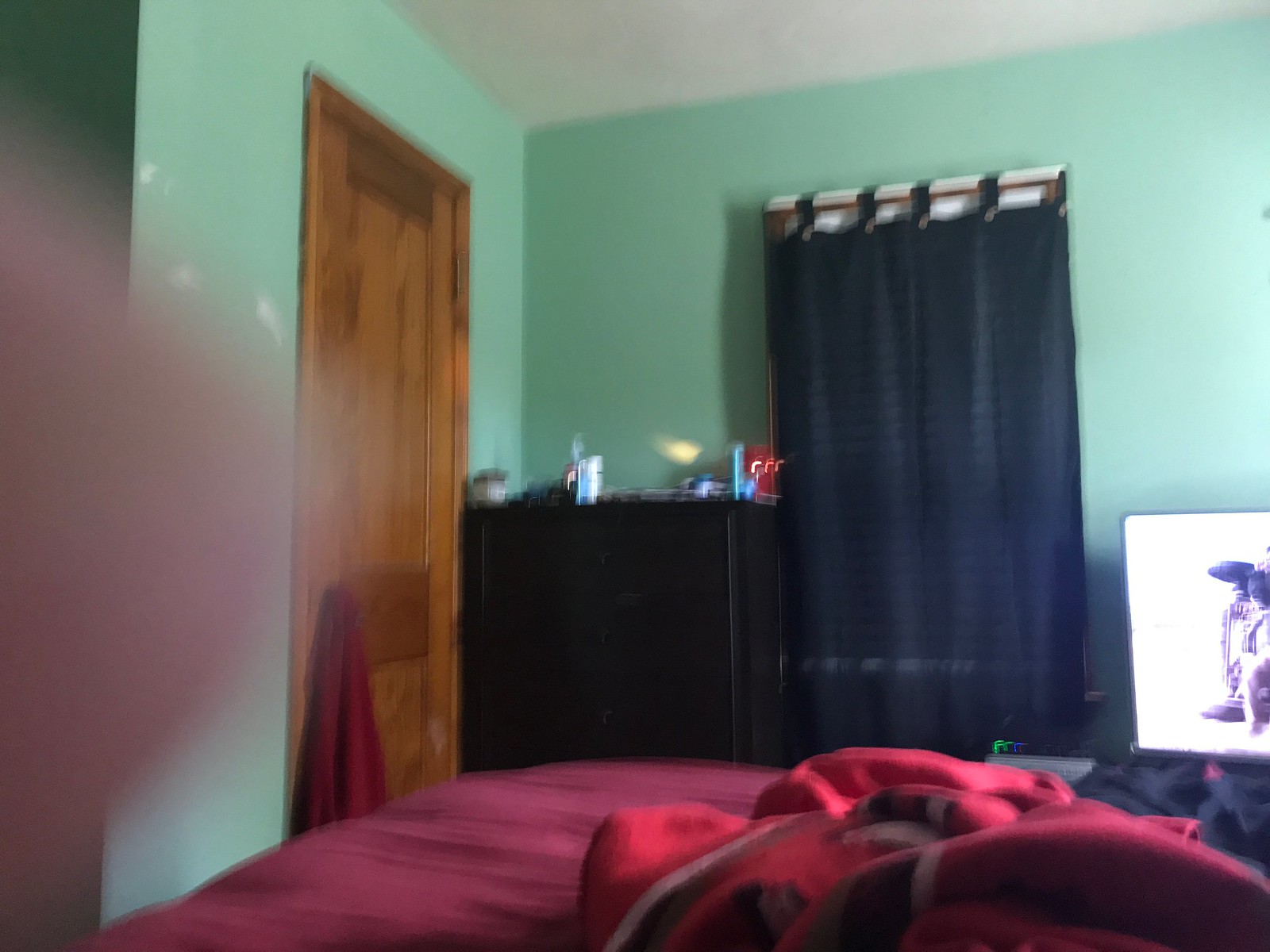A photograph captures the left side of a bedroom. Dominating the scene is an unmade bed adorned with red sheets, a matching red comforter, and a black blanket haphazardly thrown atop. The walls, painted a vibrant minty aqua, provide a refreshing backdrop. A window draped with a single black tabbed curtain allows light to filter through. A dresser is positioned in the corner of the room. To the right, a mysterious image is displayed on what appears to be a computer or TV screen, although the details of the image are indiscernible. On the left wall, a wooden door, leading to an unknown location, has a red towel casually hanging from its handle.